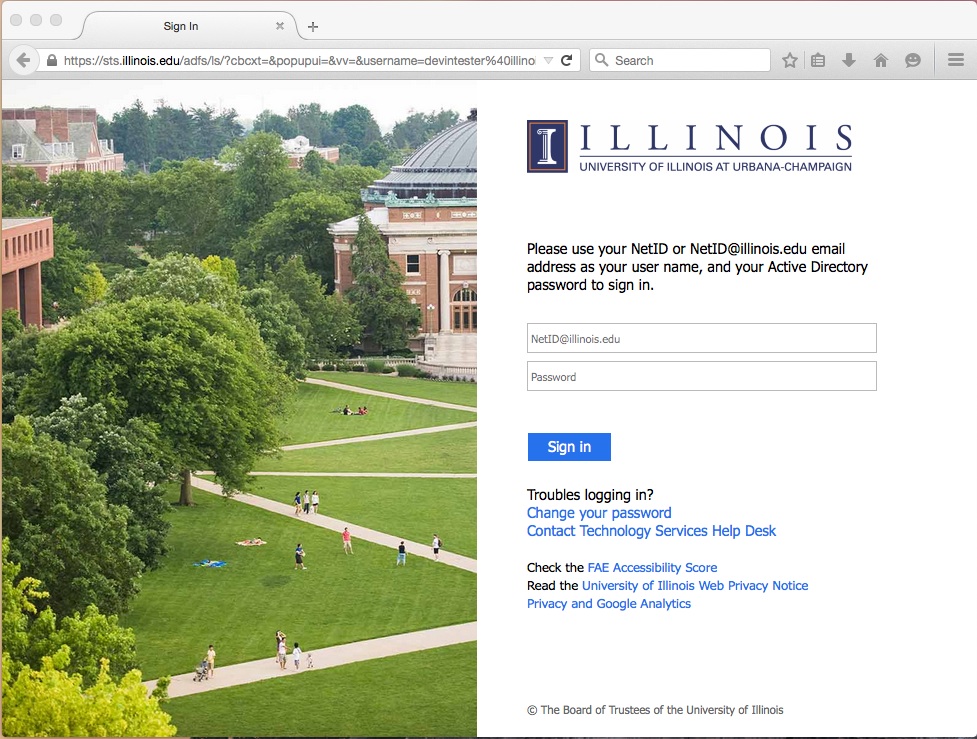A screenshot of a web login page for the University of Illinois at Urbana-Champaign is displayed on a PC monitor. The top half of the page features a picturesque photograph of the campus, highlighting numerous educational buildings surrounded by meticulously trimmed trees and a neatly mowed quadrangle intersected by sidewalks. Below the image, in darker navy blue print on a white background, is text instructing users to sign in. The instructions state: "Please use your NetID or NetID@illinois.edu email address as your username, and your Active Directory password to sign in." 

Below this, there are fields for users to input their username and password. Beneath the login fields, there is a blue "Sign In" button in white text. Additional clickable options include "Troubles logging in?", "Change your password", and "Contact Technology Services Help Desk". 

Further down, accessibility and privacy information is provided in a combination of black and blue text, including links to "Check the FAE Accessibility Score" and "Read the University of Illinois Web Privacy Notice". At the very bottom, the page includes a copyright notice: "© The Board of Trustees of the University of Illinois."